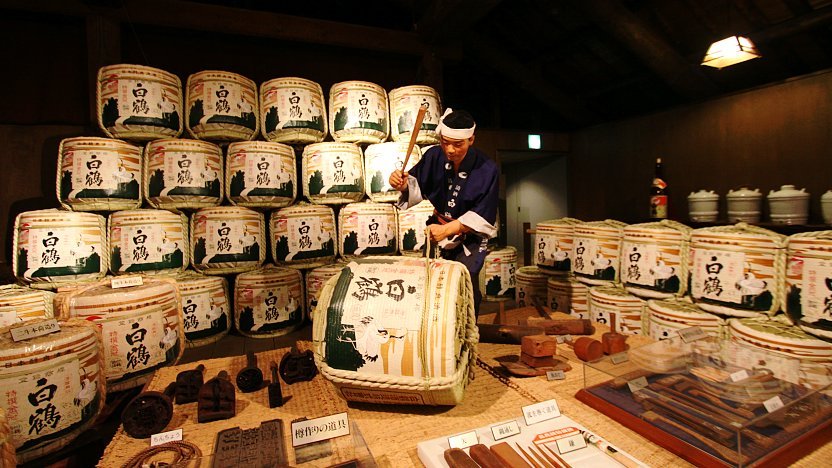The image captures an Asian-themed scene, likely a Japanese storeroom or shop, filled with culturally significant items, including stacks of barrels adorned with Japanese text and possibly sake branding. The central focus is a man, McGleng or Heck, dressed in a traditional blue kimono-like outfit and a white headband, kneeling on a carpet or mat. He is intensely working on one of the barrels, which is wrapped in rope, perhaps removing it. Surrounding him, there are four rows of five barrels each stacked on the left, with three additional ones at the bottom, and two more stacks of five barrels each on the right. These barrels, bearing Chinese characters, appear to be for sale as suggested by small price tags affixed to them. Additionally, display cases are present, containing various implements related to Japanese brewing. The setting might be part of a museum exhibit, given its detailed presentation and educational context.